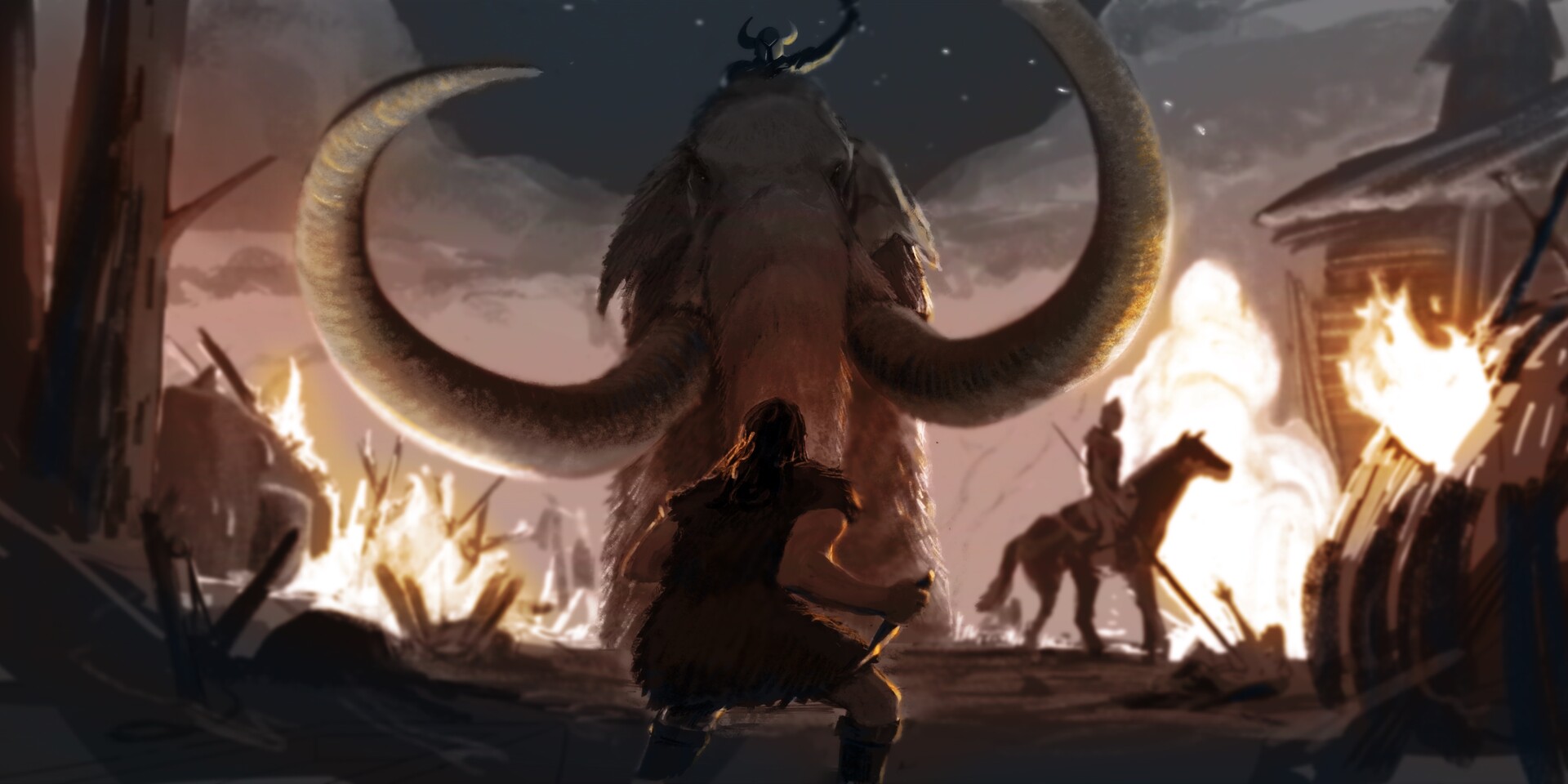The photograph presents a vivid, dynamic scene that resembles a diorama display or a moment from a video game. Central to the image is a male hunter, seen from behind, poised face-to-face with a colossal woolly mammoth. The hunter, adorned in a fur-lined shirt and trousers, and knee-high boots, clutches a dagger, ready for the confrontation. The mammoth, with its imposing, large curled tusks, looms directly at the camera, creating a moment of heightened tension. In the distance, other hunters on horseback, armed with spears, are slightly blurred, adding depth to the scene. To the left, a roaring fire suggests a strategic element to the hunt, possibly used to corner or scare the mammoth, sending plumes of smoke into a starry sky above. Above the mammoth is another figure, likely a warrior in full armor with a horned helmet, riding the beast. The background hints at a world in turmoil with raging fires and destruction, reminiscent of a prehistoric or Ice Age setting.